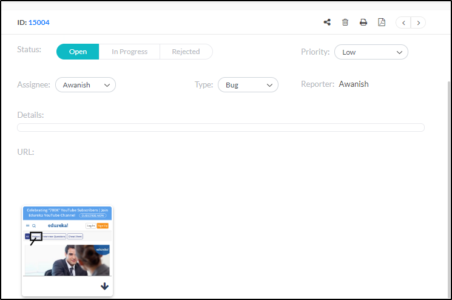ID 15004: The image showcases a user interface from a project tracking tool. At the top right corner, there's a share button located next to the ID number. Below it, there's a printer icon followed by document selectors, options for the user to configure. The interface has a section displaying the status of tasks, with a color indicator where green signifies 'Open', a task that is currently in progress or has been rejected. Additional information includes the priority being set to low, the assignee and reporter both being Awanish, and the type of task marked as a bug.

The image also includes visual elements: a blue header at the top, followed by white spaces with various geometric shapes such as squares and rectangles in black. There is an illustration of a person, a woman, and a white bottle. An arrow pointing downwards is present, outlined by a thick black border. The overall design of the website appears to be quite simple, with the 'Open' status prominently highlighted in green.